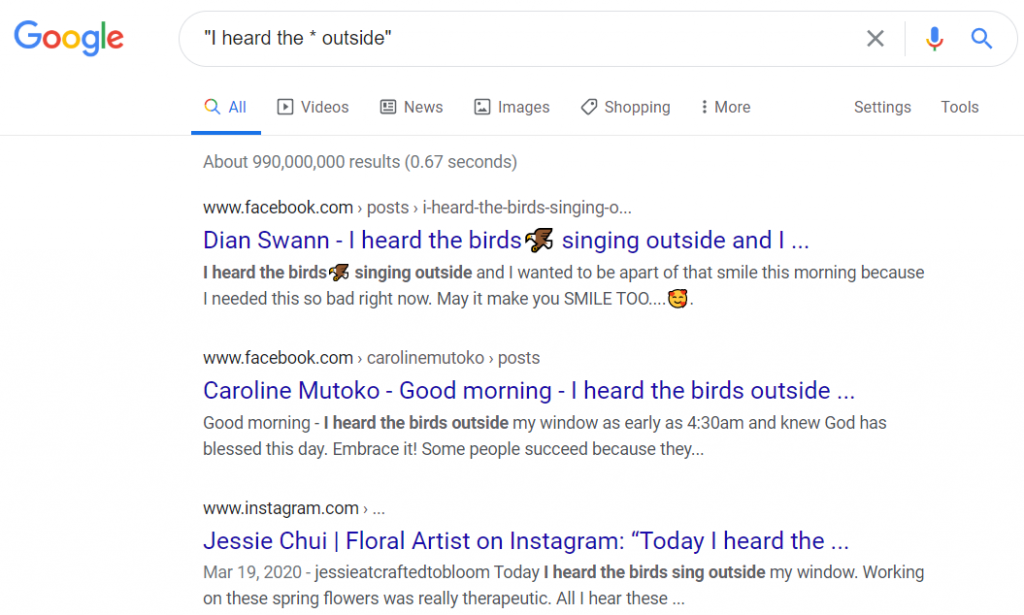The image depicts a Google search results page. In the upper left corner, the iconic multicolored Google logo is prominently displayed. Below the logo, there is a blank space, which seamlessly transitions into a search bar to the right. Inside the search bar, the query "I heard the*" is entered, enclosed within quotation marks. Directly beneath the search bar, the search tabs are visible, including options: All, Videos, News, Images, Shopping, More, Settings, and Tools.

The search has yielded approximately 999 million results in just 0.67 seconds. The first result is from a Facebook post by Diane Swan, which reads: "I heard the birds singing outside. I wanted to be a part of that smile this morning because I needed this so bad right now. May it make you smile too 😊." An icon of a bird accompanies the text.

The second result is another Facebook post, this time by Caroline Matuko. It says: "Good morning. I heard the birds outside my window as early as 4:30 AM. I knew God had blessed this day. Embrace it. Some people succeed because they..." The post trails off here, leaving the rest of the message to the reader's imagination.

The third result is an Instagram post by Jessie Chu, a floral artist. Dated March 19, 2020, the post begins, "Today I heard the..." and is captioned with: "Today I heard the birds sing outside my window. Working on the spring flowers was really therapeutic. All I hear are these..." The Instagram handle "Jessie craft the bloom" indicates the artistic focus of the poster.

Overall, the search results highlight various social media posts where individuals share their experiences of hearing birds singing outside, reflecting moments of tranquility and inspiration drawn from nature.